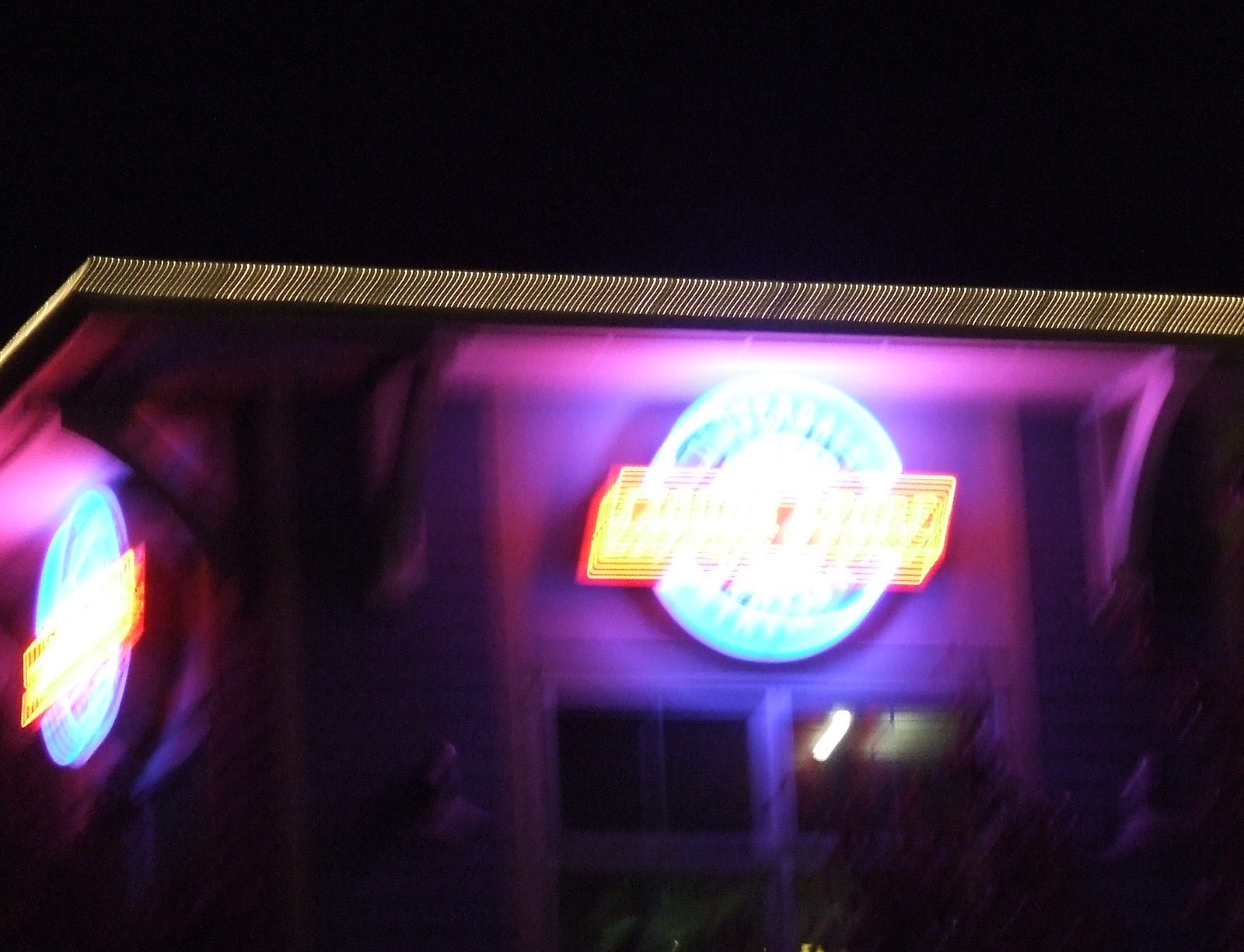This image showcases an exterior view of a building at night, though the top portion and the signage appear blurred. The prominent feature is a circular sign on the left-hand side of the building, marked by a gradient of light blue and white. Adjacent to it, a rectangular sign displays a name illuminated with yellow lights, surrounded by a red border. Both signs are accentuated by blue and purple lighting, giving an organized and aesthetic appeal.

The building's facade is clad in dark gray siding, with a window situated directly beneath the front sign. Silhouetted against the building, a couple of trees stand at the bottom and right-hand side, adding a touch of nature to the urban scene. Higher up, a series of indistinct white and gold lights blur together, creating an impressionistic effect. The backdrop is a stark black night sky, drawing attention to the illuminated elements of the structure.